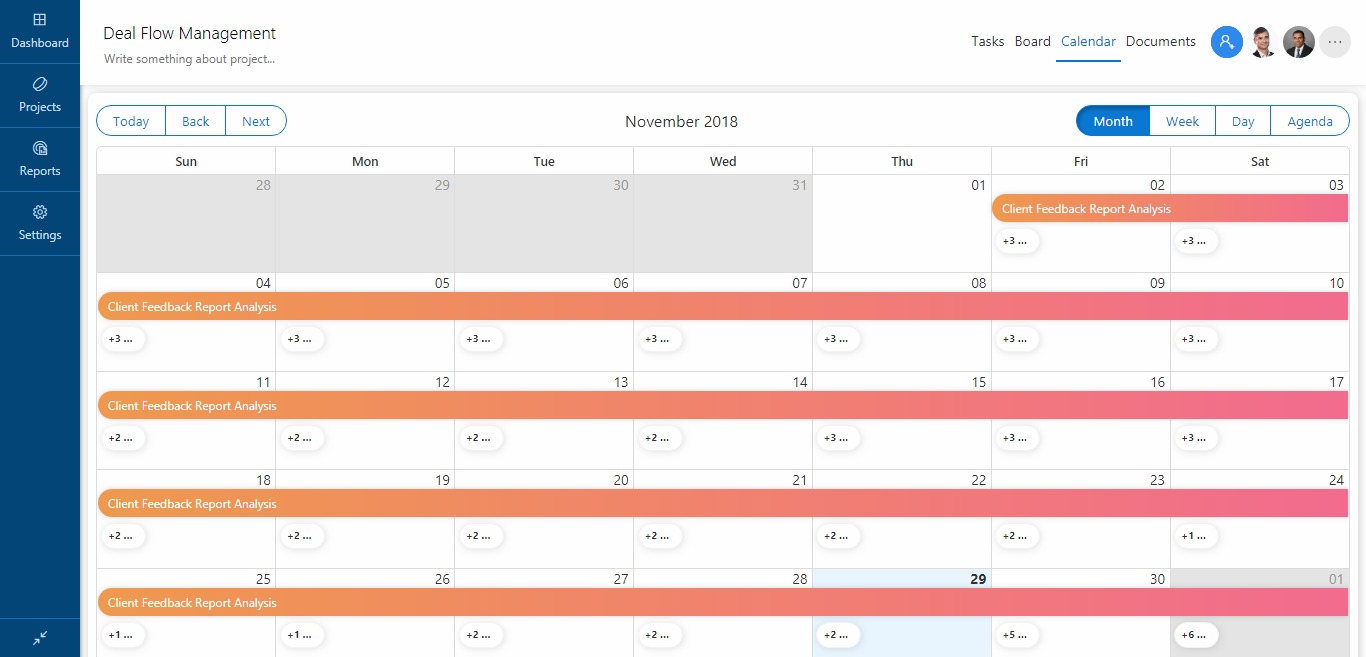The image is a detailed screenshot of a shared calendar interface, specifically showing the calendar for November 2018. The interface is part of a deal flow management system. 

In the top left-hand corner, a long vertical blue box provides various menu options including:
- **Dashboard**: Represented by a two-by-two grid icon.
- **Projects**: Illustrated with an icon resembling a yo-yo.
- **Reports**: Indicated by a circle with a document icon.
- **Settings**: Marked by a gear icon.

Directly above the calendar interface, there are additional menu options for:
- **Tasks**
- **Board**
- **Calendars** (Currently selected and highlighted in blue)
- **Documents**

To the right side of the top bar, headshots of team members who have access to and possibly are currently viewing the calendar are displayed. 

Navigation options are situated on both sides, with buttons for "Today," "Back," and "Next" located on the left, and view options for "Month," "Week," "Day," and "Agenda" on the right. The "Month" view is currently selected, highlighted in blue. 

The calendar itself is predominantly white, with certain dates grayed out:
- The first week displays grayed-out dates from October 28th (Sunday) through October 31st (Wednesday), and again for December 1st (Saturday).
- Starting from November 1st (Thursday), regular dates resume and the calendar progresses through the month.

An ongoing event titled "Client Feedback Report Analysis" is prominently highlighted in pink and orange, spanning from November 2nd to November 1st (indicating an extended period, possibly a recurring or continuous task).